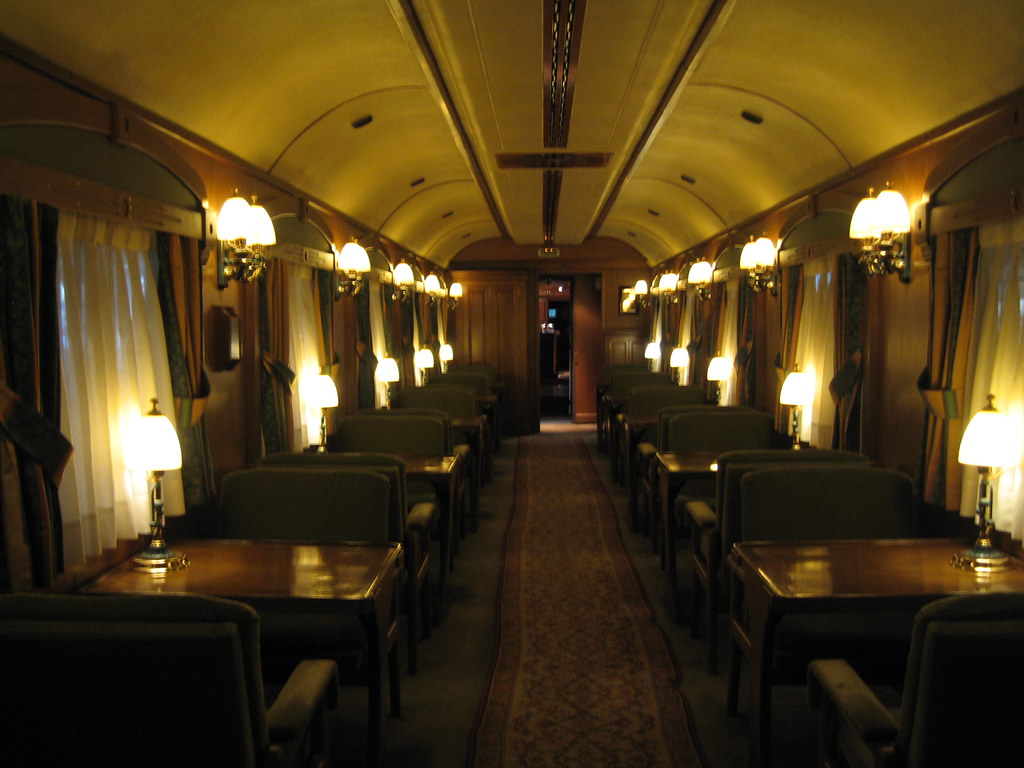The image depicts the opulent interior of a luxury train dining car, reminiscent of those found on the Orient Express. The space is adorned with rich, dark wood paneling and features a series of elegant tables, each flanked by two plush chairs. The ceiling arches into a polished dome with intricate detailing, contributing to a sophisticated ambiance. Above each table, dual lamps with gold bases and white shades cast a warm glow, though the overall lighting remains subdued, enhancing the car's intimate, upscale feel. Large windows with sheer curtains and draped brown curtains stretch along the walls, spaced a few feet apart, providing glimpses of the outside world. A burgundy runner elegantly divides the car's floor, adding a touch of grandeur. At either end of the dining car, wooden sliding doors enhance the space’s luxurious appeal. The entire setting exudes a nostalgic charm, evocative of a bygone era of opulent train travel.